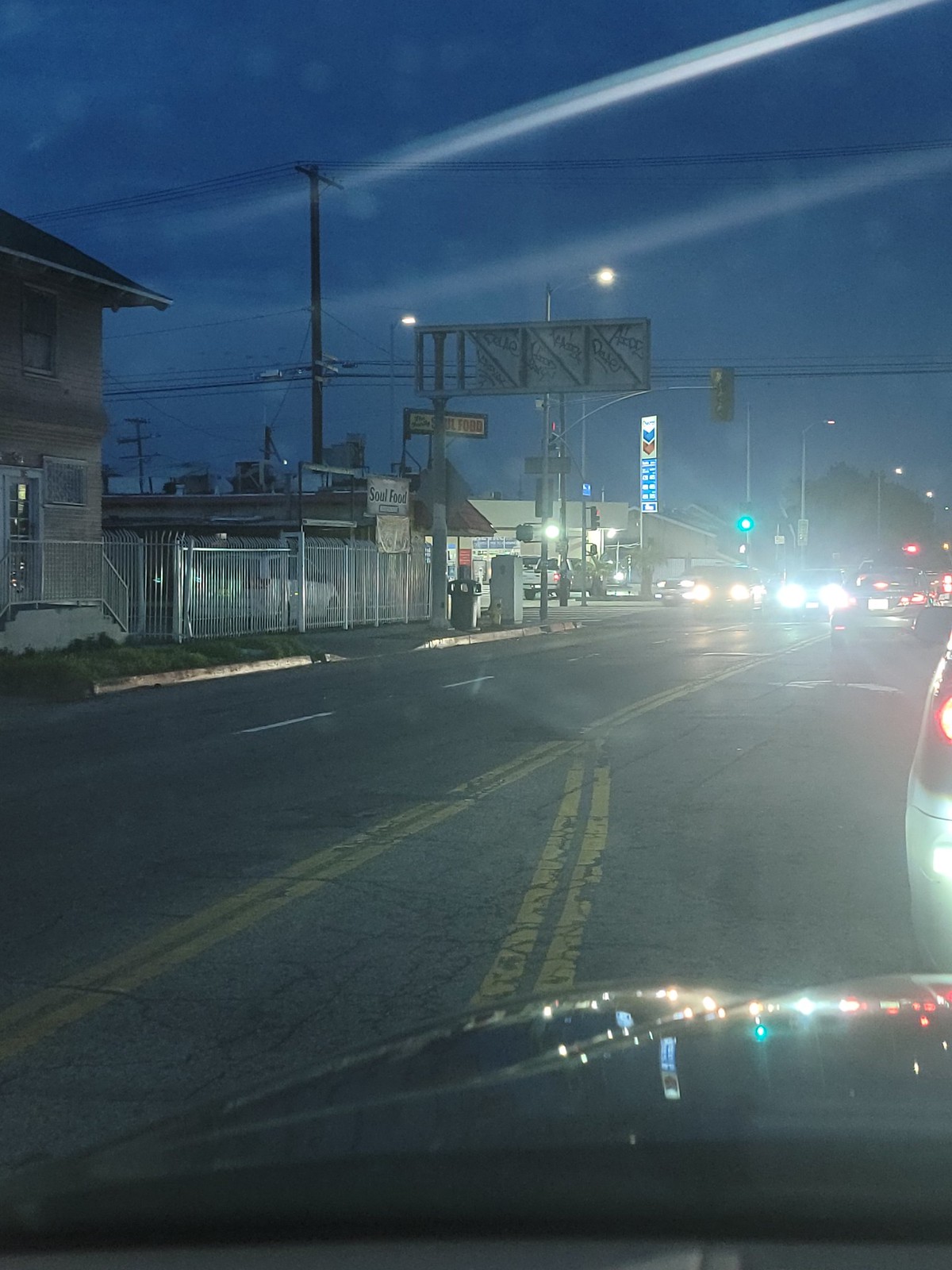A nighttime street view photographed from inside a car, revealing the scene through the windshield, with the car's hood prominently visible at the bottom. The hood reflects the glimmer of headlights, a green traffic light, and some red stoplights, adding vibrant colors to the image. Directly ahead, the back bumper of a white car with illuminated red taillights is clearly visible. The street is marked by dual yellow solid lines running down the center, while oncoming cars with bright white headlights approach on the opposite side.

In the distance, the sky is dark, punctuated by two small, glowing dots, likely streetlights. On the left side of the image stands a building bordered by a metal fence. Further down the road, a brightly lit gas station can be seen, characterized by a long rectangular sign. The sign features a white top section with blue and red bands and a blue area displaying gas prices. Adding to the urban landscape, both a green and a red traffic light are visible in the distance.